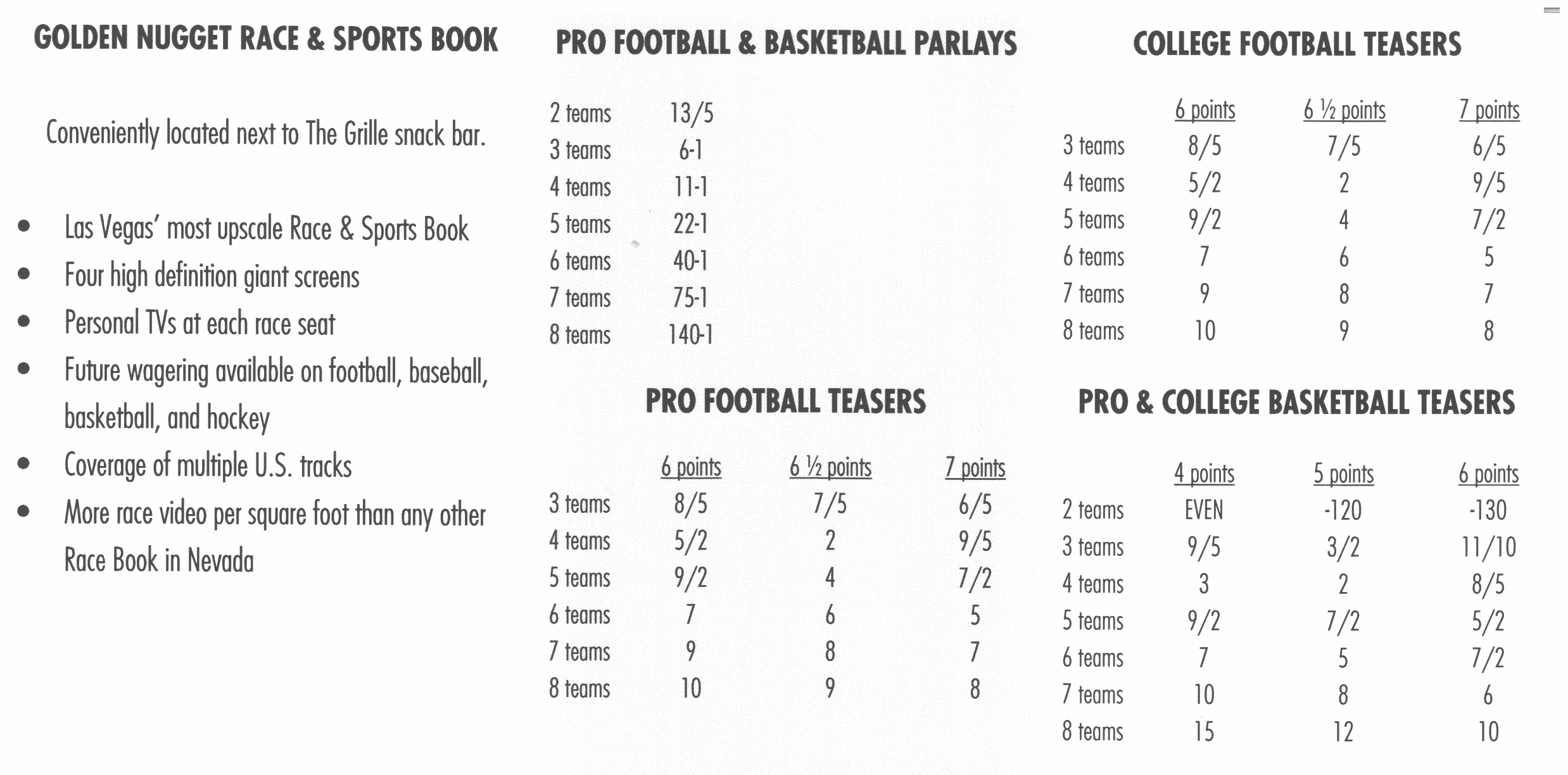This horizontal rectangular image, with no border, is a black and white text-only display that details a betting book from Golden Nugget Race and Sportsbook. The upper left section prominently features the title "Golden Nugget Race and Sportsbook" in larger font, followed by several bullet points. These bullet points highlight its various offerings: it is conveniently located next to the Grill Snack Bar and is touted as Las Vegas's most upscale race and sportsbook. The amenities include four high-definition giant screens, personal TVs at each seat, future wagering on football, baseball, basketball, and hockey, coverage of multiple U.S. tracks, and more race video per square foot than any other race book in Nevada. On the right side of the image, four sections provide detailed sports betting information under dark-lettered headings: "Pro Football and Basketball Parlays," "College Football Teasers," "Pro Football Teasers," and "Pro and College Basketball Teasers." These sections outline the odds based on the number of wins, tailored for different betting scenarios.